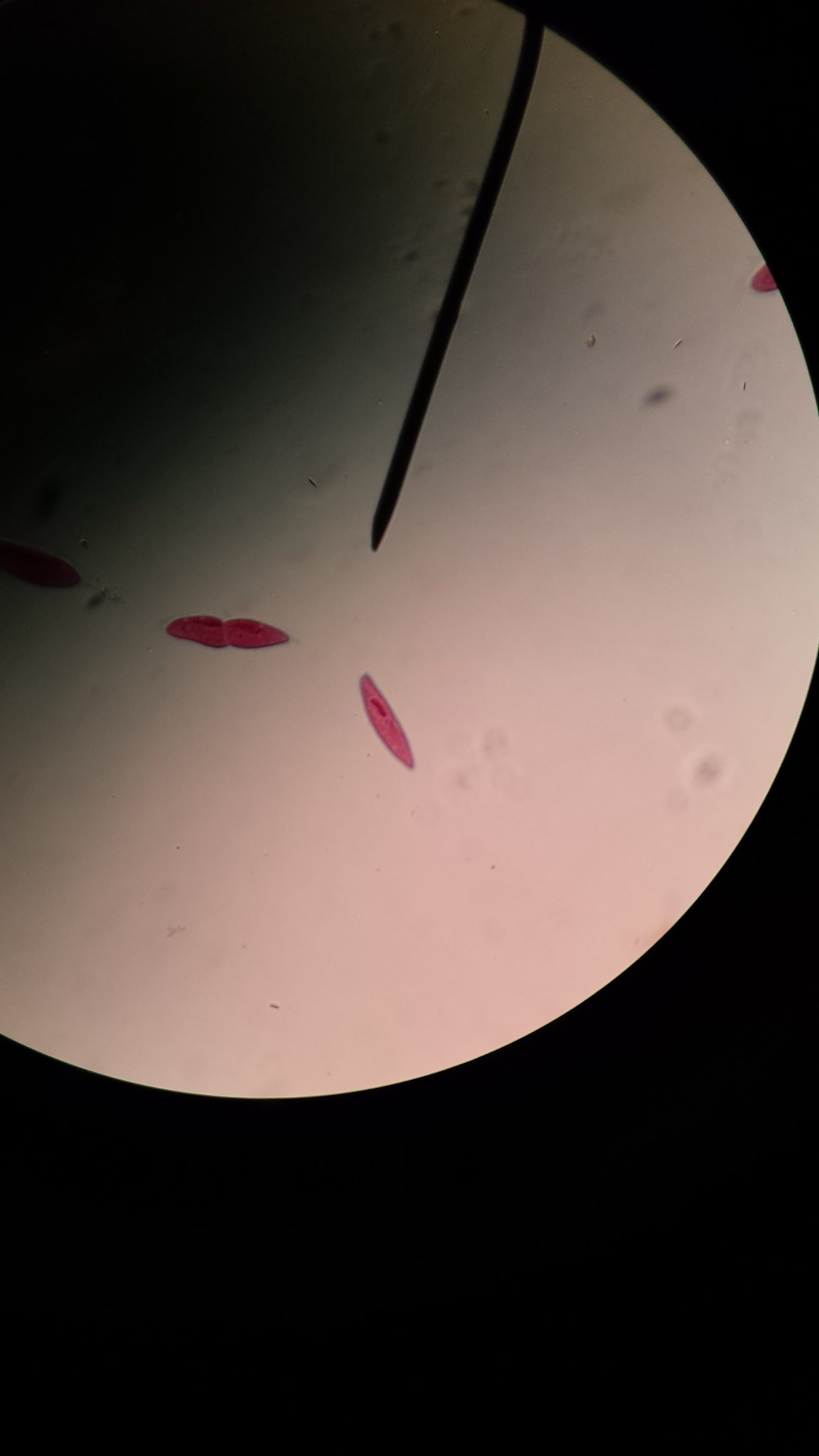The image is an abstract composition dominated by a pitch-black background. In the upper section, extending slightly lower, there's a large, partially obscured white disc reminiscent of the moon. This disc has a waxy, cheesy texture, with surface imperfections resembling tears or stretches, some of which appear purple. A prominent dark line or band bisects the circle, adding a sense of division. Additionally, there are sporadic red streaks across the disc, contributing to its mysterious and otherworldly appearance. The image is devoid of text, emphasizing its enigmatic and interpretative nature.